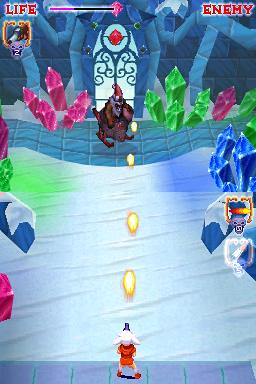In the image, the top left corner features a red section labeled "Life," accompanied by a life bar. To the right, there's a purple bar with text in black and purple colors. The top right corner has a red section labeled "Enemy." Below this, there's a symbol resembling a shotgun or gun with the number "2" underneath it, indicated by an orange bar. 

At the center of the image, an archway dominates the scene, topped with a red diamond and surrounded by curly patterns within a circular design. The background features a blue wall, with pink crystals on the left and green crystals on the right. Additionally, there's a red crystal present, and the ground consists of blue tiling.

At the bottom of the image, a character is depicted shooting yellow orb-like bullets towards a creature. This character has distinctive white ears, an orange tunic, yellow pants, and red shoes, standing on tiling amidst a sandy area that resembles white sand. The environment also includes blue crystals to the right and green crystals to the left.